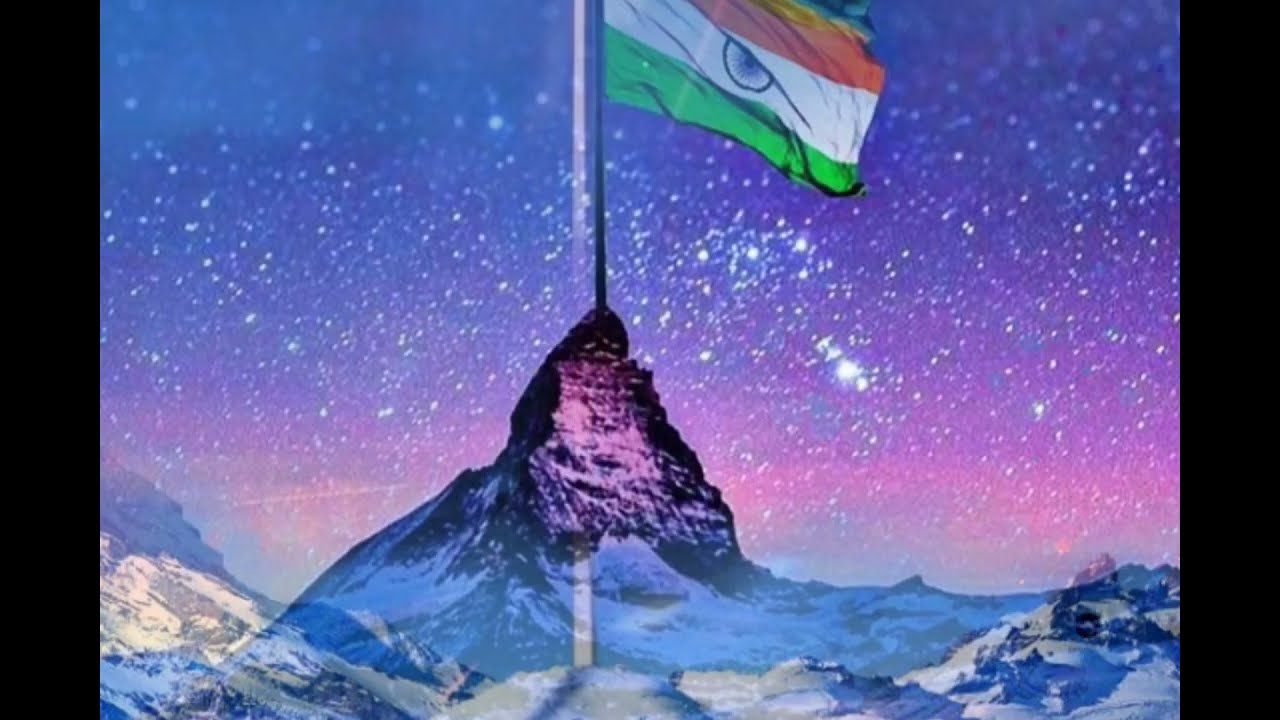This digital artwork depicts a scenic mountain landscape enveloped in snow, set against a vivid, multi-hued sky. The mountain range occupies the bottom 25% of the image, with a notable peak rising prominently at the center, accentuated by lavender and black tones with snowy patches. A flagpole runs vertically from the base of the mountain to the top, seemingly superimposed onto the scene; it features a multicolored design with blue, yellow, red, white, and green stripes, adorned with an eye symbol—a black iris encircled by a blue ring. The sky transitions from deep blue at the top to violet and then to white near the horizon, peppered with snowflakes that resemble stars, creating a celestial atmosphere. This artistic rendering captures the grandeur of a snow-clad mountain valley, bathed in the surreal glow of an evening sky.